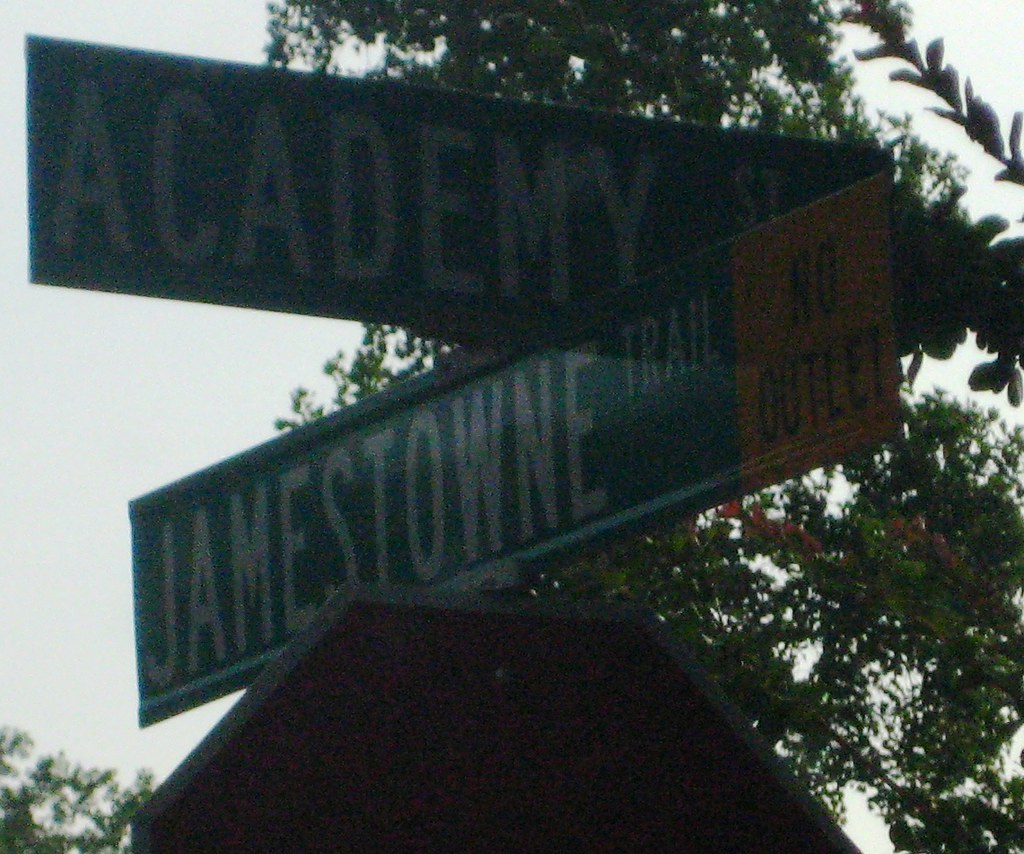In this dimly lit photograph, two road signs stand at a junction, indicating a crossroads. The signs, painted in traditional green with white lettering, bear the names "Jamestown Trail" and "Academy Street." A bright yellow "No Outlet" notice is appended to the end of the Jamestown Trail sign. Positioned atop or just behind a partially visible stop sign, these directional indicators are the only clear elements in the shadowy scene. The backdrop features dense tree foliage, primarily green with splashes of orange, suggesting a shift in seasons. The sky overhead is a very pale blue, hinting at dusk as the likely cause of the subdued lighting. The arrangement of the signs, one above the other and pointing in different directions, unequivocally marks this as an intersection.